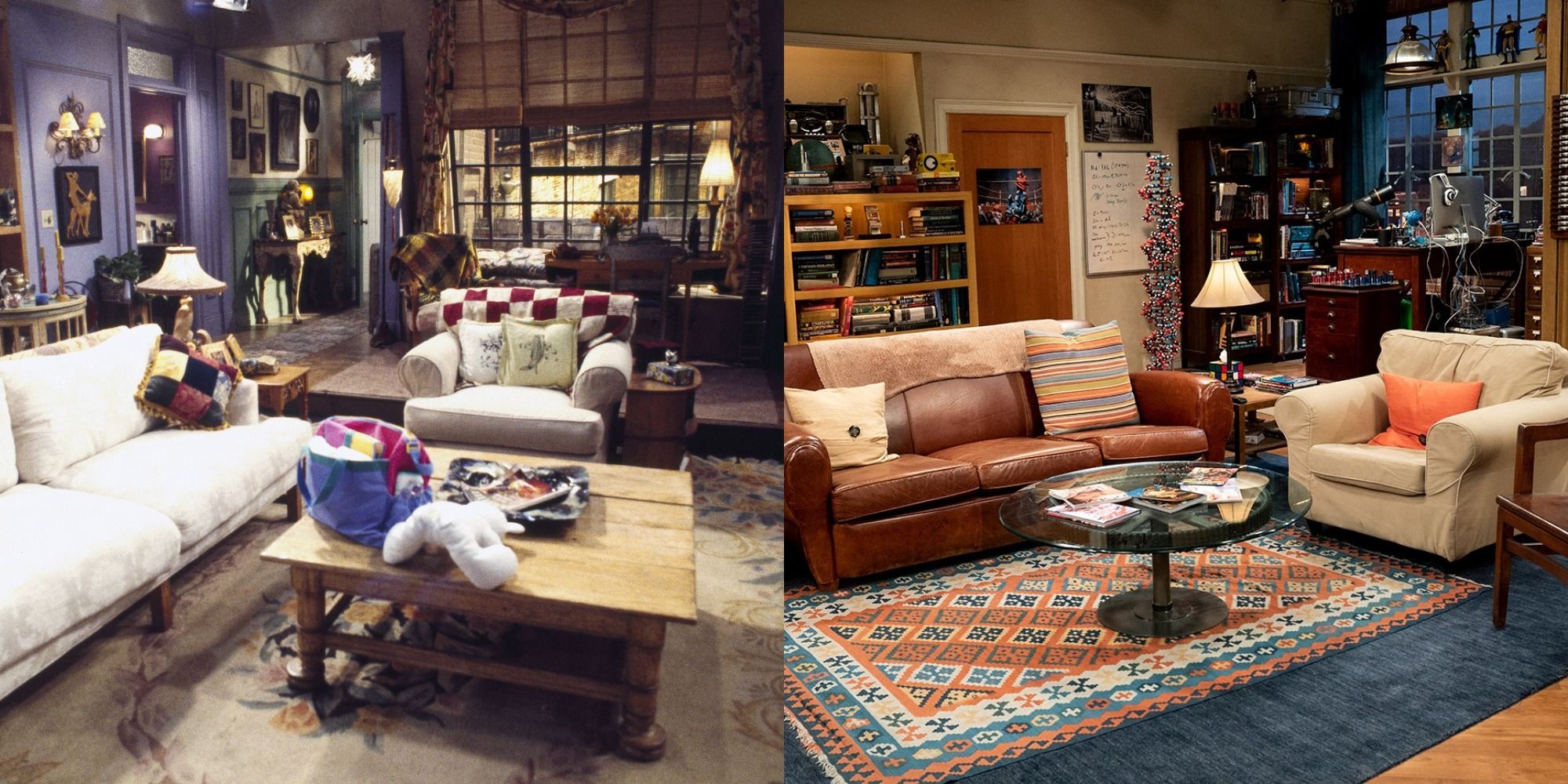This is a split-combination photo showcasing two intricately decorated seating areas, each reminiscent of a television studio, particularly the show "Friends." On the left, the seating area features deep purple walls and a white couch complemented by a big square wooden table that holds some knitting supplies. A large stuffed chair and pretty ceiling lights hang down, giving it a more formal setting. The floor hosts a throw rug, and above it sits a white couch adorned with a checkered blue, black, red, and yellow pillow. A lamp hovers above the couch, casting a warm light.

To the right, the decor contrasts with a country-style look. The walls are blue and lined with pictures, leading to a big multi-pane window with brown shades halfway up. In front of the window, a reddish-brown leather sofa is positioned next to a light beige chair with an orange pillow. The scene is grounded with a solid blue rug layered with another rug featuring orange, blue, and white edges. Between the seating is a central oval table on a blue, white, yellow, and red print throw rug, which holds various pamphlets or books. A telescope, bookcase, and an assortment of books and albums fill the background, reinforcing the busyness of the room. Overall, both rooms feature a combination of variously colored couches, eclectic furnishings, and a blend of modern and country aesthetics.